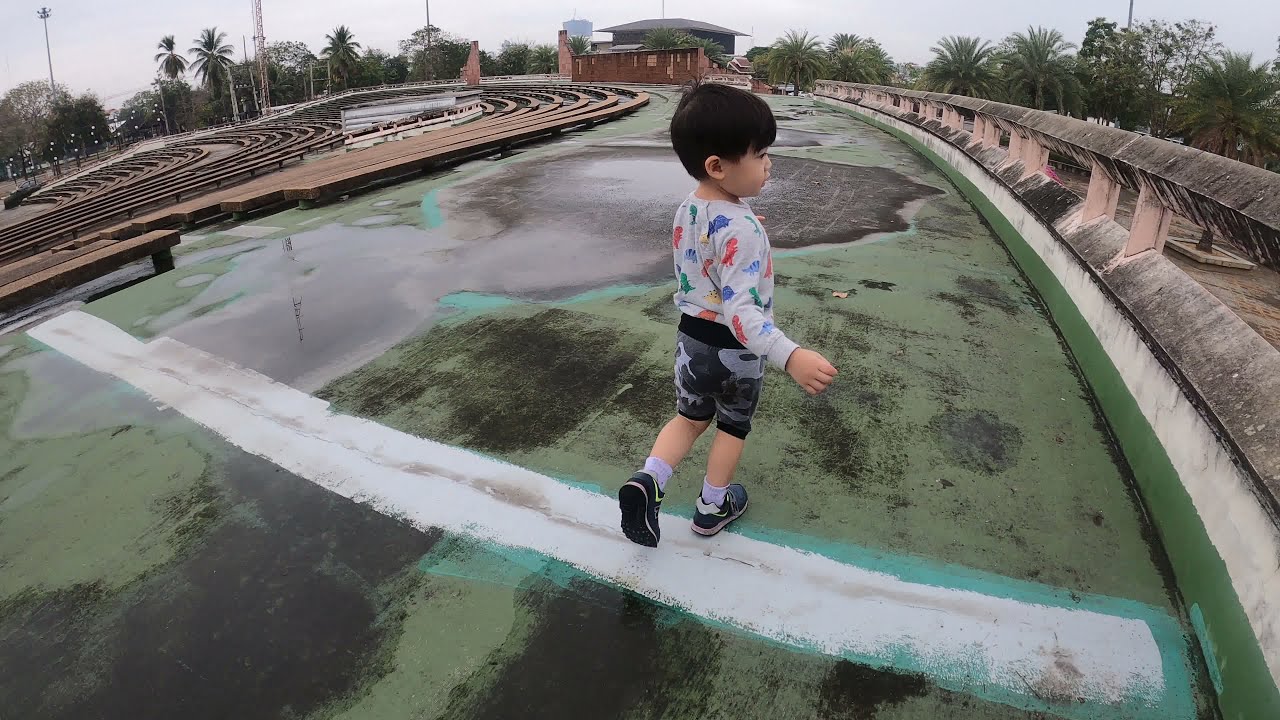The photograph captures a young Asian boy, approximately four or five years old, walking along a green, dirty, and perhaps moldy-looking track or walkway adorned with white stripes. His outfit features gray camouflage shorts, and a mostly white shirt decorated with colorful dinosaur prints. He sports dark bluish, yellow, and white sneakers. The scene appears to be in an outdoor setting that resembles a smaller-scale Olympic Coliseum or amphitheater with a stone guardrail to his right and stone benches on his left. The background includes palm trees, a brownstone building, and additional structures, all under a gray sky. The surrounding appearance is dismal and weathered, possibly indicating recent rainfall given the presence of rain puddles.